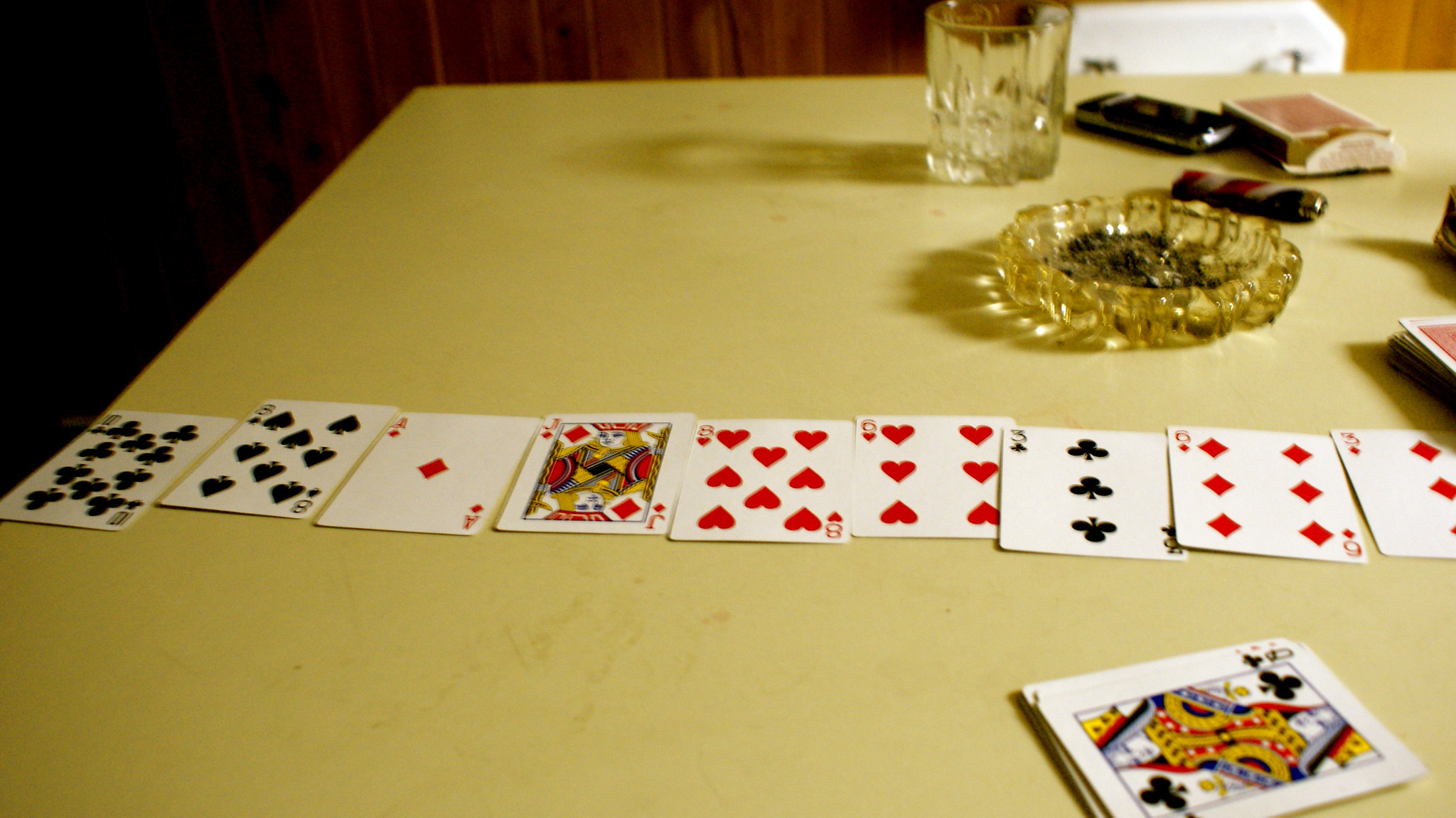The image depicts a pale yellow card table, possibly a card table, with various playing cards and accessories arranged across its surface. At the lower right of the table, there is a stack of cards with the queen of clubs visible on top. Spread horizontally across the middle of the table are the nine of clubs, seven of spades, ace of diamonds, jack of diamonds, eight of hearts, six of hearts, three of clubs, six of diamonds, and three of diamonds. Above these cards is a clear glass ashtray containing ashes, flanked by two lighters. To the right, additional playing cards are scattered. Positioned towards the upper part of the image is a clear glass. The upper left corner of the image is quite dark, contrasting with the wooden wall stretching across the background. The right side of this wall is brightly lit, though partially obscured by a white object at the top. To the left of the glass and ashtray, shadows are cast, adding depth to the scene. The layout also includes an open box for the playing cards.